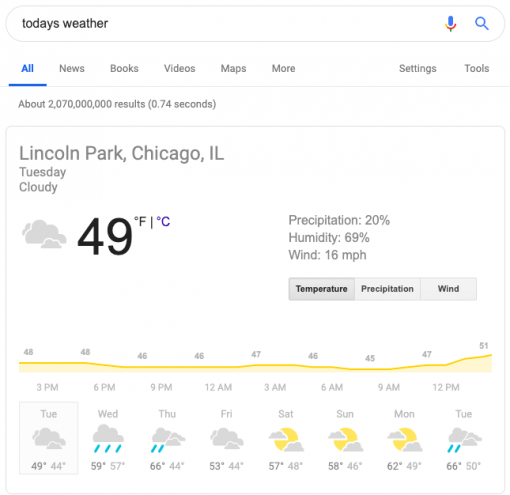**Caption:**

This screenshot showcases a search results page with a focus on the day’s weather information. The background is pure white, creating a clean and uncluttered visual. At the top of the page, there's a search bar designed in an elongated pill shape with a light gray outline, containing the text "today's weather." Below the search bar, a navigation menu features various options. The "All" option on the left is highlighted in blue text with a blue underline, while to its right, options such as "News," "Books," "Videos," "Maps," "More," and then "Settings" and "Tools" at the far right are displayed in gray text.

Directly beneath the menu, a light gray line separates it from the search results. An informational line states, "About 2,070,000,000 results (0.74 seconds)." The first result is a weather information card, bordered by a thin gray line with rounded corners. On the top left of the card, it states "Lincoln Park, Chicago, Illinois," followed by "Tuesday" and a "Cloudy" label next to an image of clouds. The temperature is presented as "49°F," with an option to switch to Celsius in purple text, though it is not currently selected. On the right, key weather metrics are provided: "Precipitation: 20%," "Humidity: 69%," and "Wind: 16 mph."

Below this summary, three gray buttons allow for further interaction. The slightly darker button marked "Temperature" is selected, while the other two options are "Precipitation" and "Wind." The card continues with a graphical representation of the temperature throughout the day and a seven-day forecast. Tuesday is highlighted as the selected day, enclosed in a gray box, showing temperatures with a cloud icon: "49°F" in darker text and "44°F" in lighter text. Next to Tuesday, the forecast for Wednesday is displayed with a rain cloud icon and temperatures "59°F" in darker text and "57°F" in lighter text.